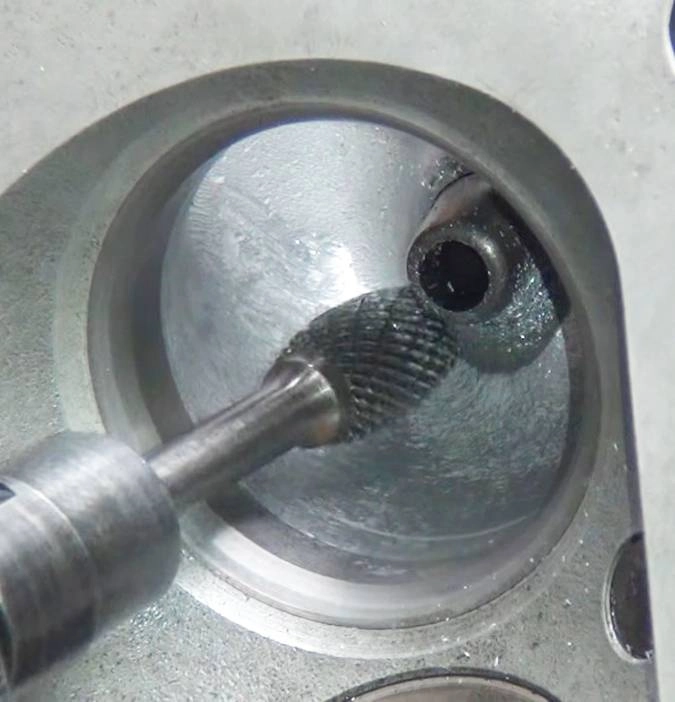This close-up color photograph focuses on a silver automobile part that prominently features a round hole. The metal piece has a thick rim with a recessed, shiny interior that has been meticulously smoothed out. Attached to a metal drill, there is a wire brush where a drill bit would typically be, indicating the tool's purpose in cleaning and grinding the hole. The process has left behind scattered metal shavings both inside the hole and on the surrounding surface, emphasizing the precision work involved. The background includes elements that suggest the part is situated within a vehicle, with hints of car paint visible, adding context to the meticulously refined appearance of the drilled and cleaned metal part.